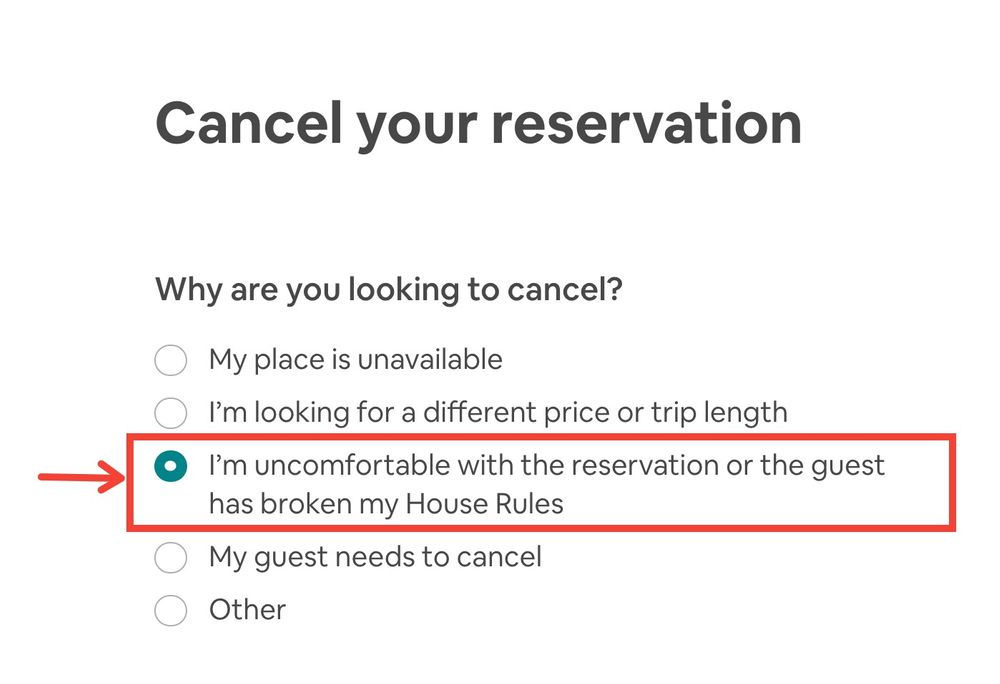Screenshot of the reservation cancellation page, likely for Airbnb, with a white background. At the top of the page, it shows the prompt "Cancel Your Reservation?" in bold black text. Below the prompt, a question asks, "Why are you looking to cancel?" followed by a list of five options for cancellation reasons. Each option is accompanied by a fill-in bubble:

1. My place is unavailable.
2. I'm looking for a different price or trip length.
3. I’m uncomfortable with the reservation or the guest has broken my house rules. (Highlighted with a red arrow and a red box around it)
4. My guest needs to cancel.
5. Other.

All text on the page is in dark black or light gray, making it easy to read.